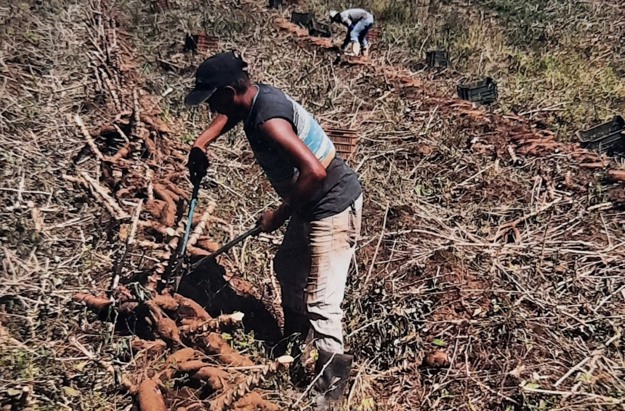A vivid photograph captures the labor-intensive process of cassava harvesting in a developing region. In the foreground, a worker is skillfully using a lopper tool—a long-handled cutter—to harvest the cassava tubers from the ground. The worker is dressed in a dark baseball cap, a short-sleeved dark shirt, and sturdy boots, underscoring the practical attire necessary for this demanding work. In the background, another worker is also visible, bent over and engaged in the same task, highlighting the collaborative effort required for this agricultural process. To the right of the image, there are piles of harvested cassava, along with baskets and totes that are likely used for transporting the tubers. The field itself shows signs of extensive activity, with visible paths where the ground has been walked and driven on, leading to a row of neatly piled cassava on the left side of the photograph. This image not only documents the physical effort involved in cassava harvesting but also emphasizes the crop's importance as a staple food in the developing world.